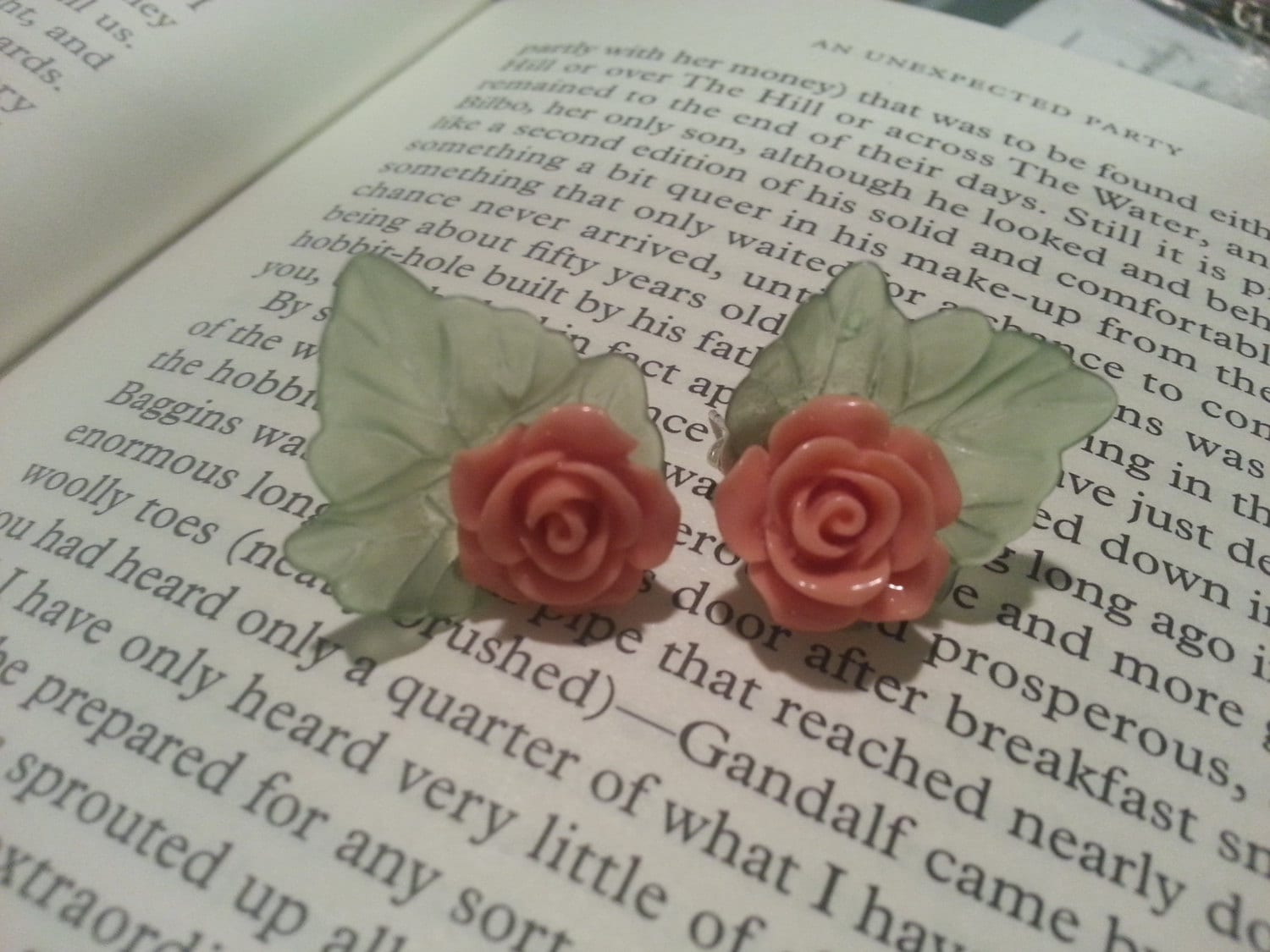The image depicts two intricately crafted objects, difficult to identify with certainty due to the angle, but they appear to be delicate rose-shaped accessories, potentially made of porcelain or clay. The roses exhibit a soft, pale pinkish-peach hue, with an artistic finish that gives them a glossy, almost translucent appearance. Each rose is backed by a wide, green leaf, enhancing their natural beauty. These items are small enough that they could be either earrings or pins. They rest gracefully atop an open book, with the heading "An Unprotected Party" visible at the top of the page, adding a touch of literary sophistication to the scene.